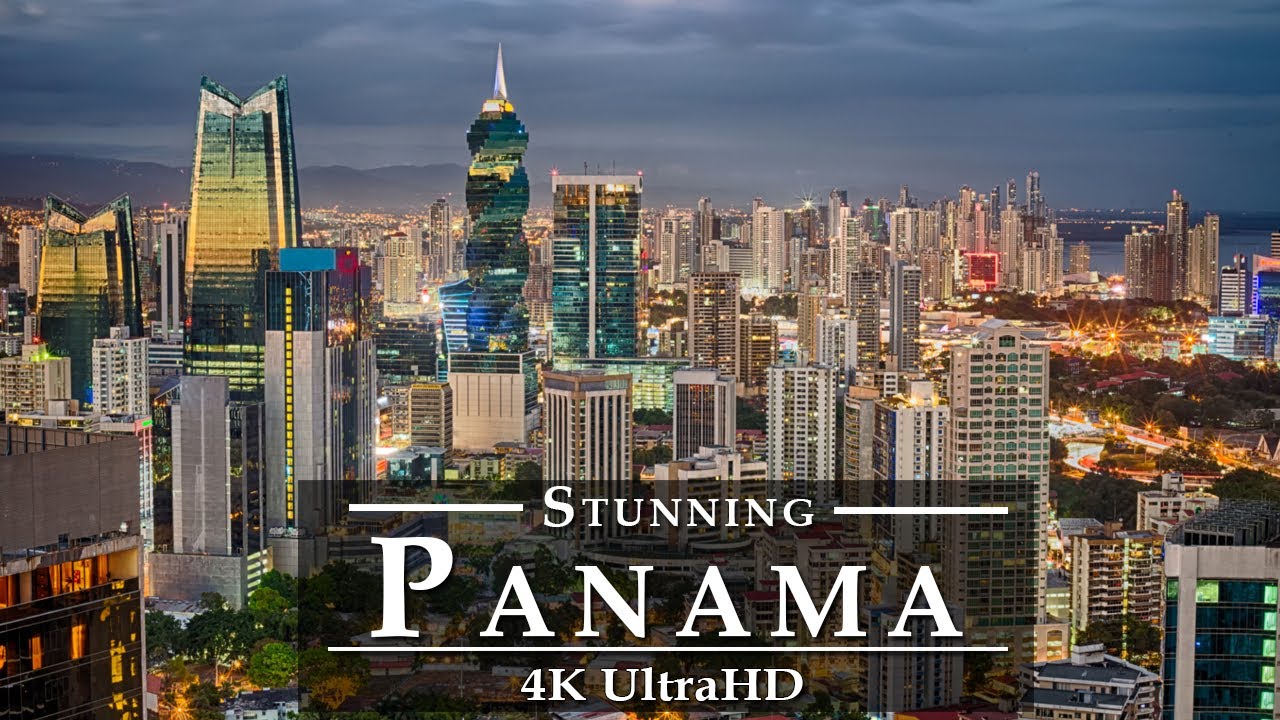This vivid color photograph captures the expansive skyline of a bustling city from a remarkable aerial perspective. Towering skyscrapers starkly contrast against a somber, overcast sky laden with thick clouds. Among the architectural marvels, two distinctive skyscrapers on the left feature mirrored facades and a unique V-shaped notch at the top. Central to the composition is an eye-catching skyscraper with a spiraled design, adding a dynamic element to the scene. 

The photograph's lower portion includes a large, semi-transparent gray rectangle overlay, which subtly reveals the buildings beneath. This overlay prominently displays the text: "STUNNING PANAMA 4K ULTRA HD." Both phrases are rendered in crisp white letters, with "STUNNING PANAMA" in all caps. The word "PANAMA" is particularly notable for its uneven kerning, most noticeably where the letter "P" is spaced unusually far from the rest of the word. Additionally, thin white lines border the "STUNNING" text on both sides, and "PANAMA" is underlined with a delicate white line. The scene is devoid of any human or animal presence, focusing solely on the intricate urban landscape.